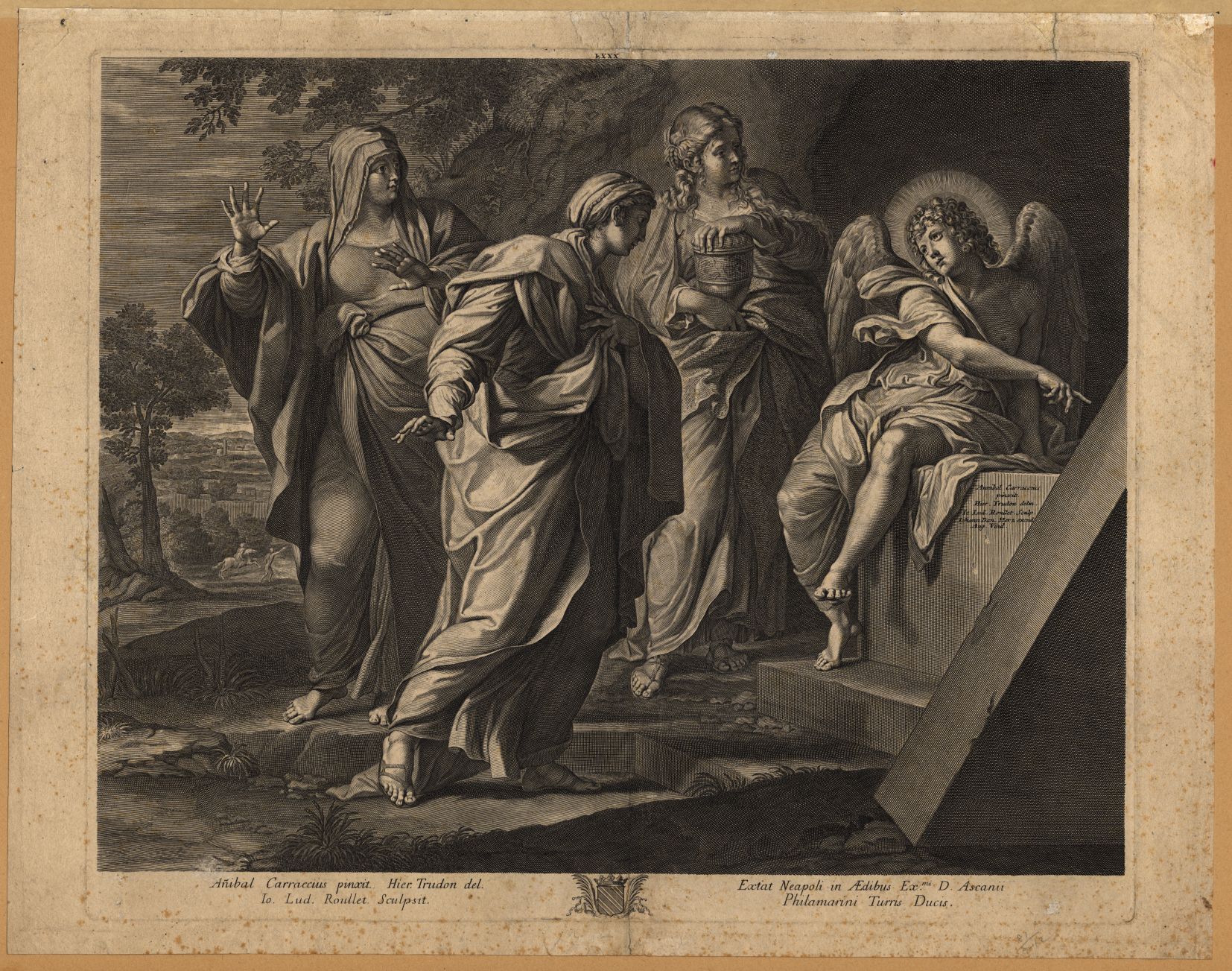The artwork is a hyper-realistic pencil and charcoal drawing on a tan or brown paper canvas, depicting a striking and intricate scene. At the center right of the composition is a cherubic angel, characterized by their curly hair, light-colored robes, and feathered wings. The angel, seated and leaning on a stone block or tombstone, points towards the right side of the image, suggesting a narrative element beyond the frame. 

To the left of the angel stand three women, all adorned in long, flowing robes. The woman closest to the angel holds a large urn and wears sandals; her long hair cascades loosely over her shoulders. Beside her, another woman, draped in similar robes with a cloth covering her hair, faces the right side of the frame, adding to the sense of attention directed towards the angel. The third woman stands with both her hands extended towards the viewer, palms outward, her head also covered with a cloth and her expression suggestive of surprise or awe.

They stand upon a rocky platform, with a rich background that includes trees, grassy land, and distant horses and people, possibly in a city or village setting. At the bottom of the image, there is text in a foreign language, written in the same color as the drawing, accompanied by a small emblem or crest. The black and white tones, combined with the brown of the paper, create a detailed and textured visual experience, emphasizing the realistic folds of fabric and intricate details of the scene.